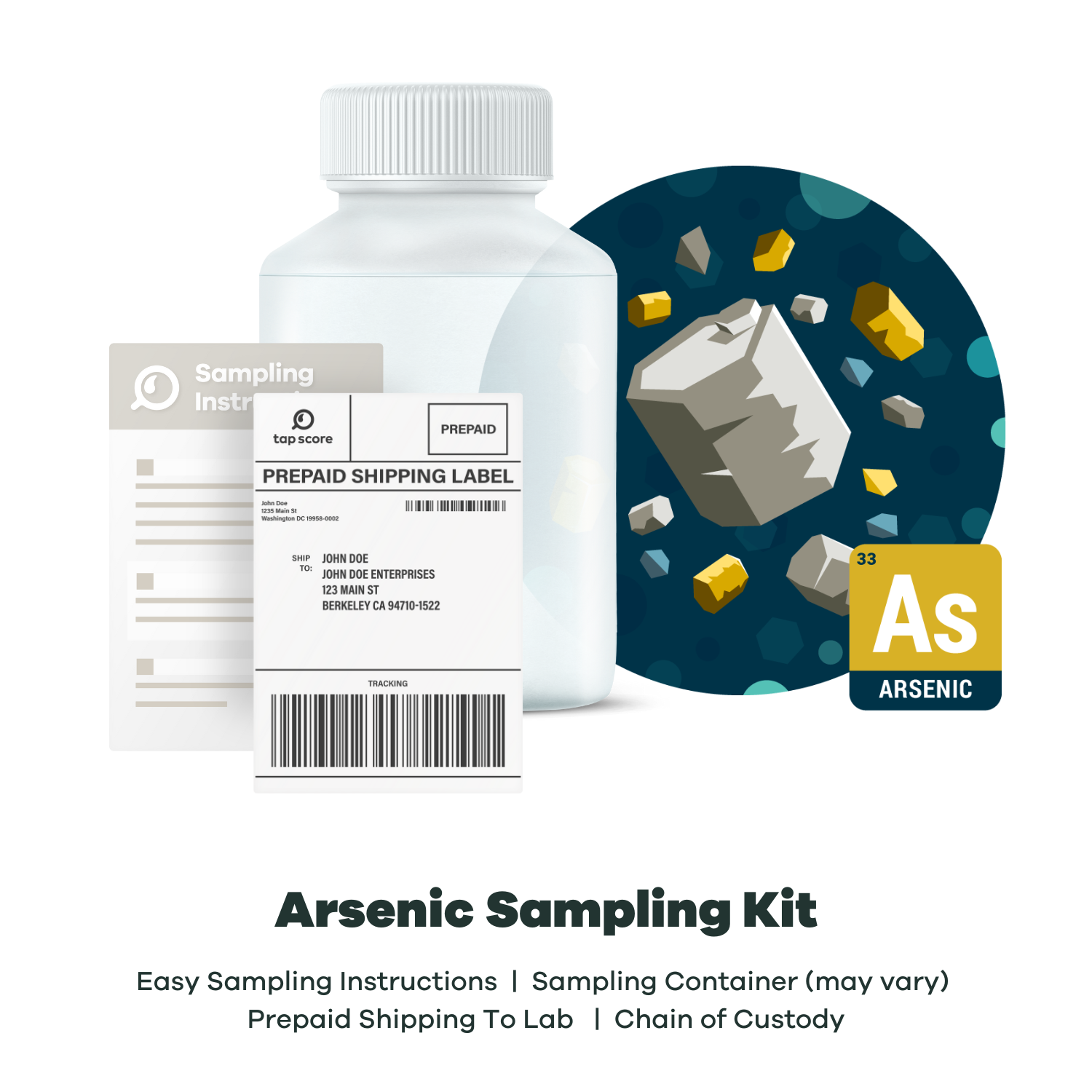The image is a computer-generated promotional graphic on a white background, depicting an arsenic sampling kit. At the bottom of the image, black text reads: "Arsenic Sampling Kit. Easy Sampling Instructions. Sampling Container. May Vary. Prepaid Shipping to Lab. Chain of Custody." Above this text is a representation of the kit's contents. 

In the center, there's a transparent or semi-transparent plastic bottle that appears to be empty or contains a clear liquid. To the left of the bottle, a prepaid shipping label with a placeholder "John Doe" address is displayed, serving as an example. Slightly further left is a rectangle titled "Sampling Instructions," which contains blank lines indicating where instructional text would be.

On the right side of the bottle, there is a colorful circular illustration featuring yellow, white, blue, and gray shapes surrounding a central gray figure. Adjacent to this, a small, square graphic mimics the periodic table entry for arsenic, marked with a yellow and black background. It displays "AS" in white text, "33" in the top left corner, and "Arsenic" beneath in smaller script. This detailed and visually informative image advertises the arsenic sampling kit, incorporating elements of graphic design to clearly present its key components and functions.